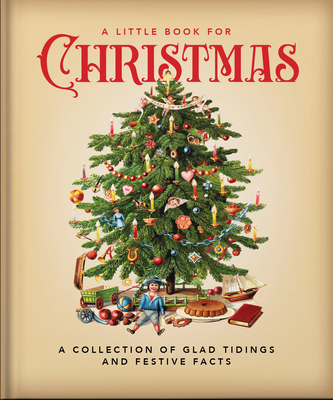The image depicts the cover of a vintage-style children's book titled "A Little Book for Christmas." The book has an aged cream or tan background with a darker gray binding. The title is written in ornate red lettering, with the word "Christmas" prominently displayed. Below the title, a short needle pine Christmas tree is decorated with old-fashioned adornments, including candles, handmade streamers, small wooden ornaments, and older style decorations such as letters and dolls. At the base of the tree, a variety of period toys and items are spread out, including an antique-style military doll, a round baked dessert, a small book, a wooden ship, a toy cannon, a little wagon, some fruit, and a cake. Additionally, a small child wearing a blue jacket, blue hat, and green pants is seated on the floor near the tree, surrounded by toys like balls and cards. The tagline at the bottom of the cover reads, "A Collection of Glad Tidings and Festive Facts," in black text. The background of the cover appears to float against a white backdrop, emphasizing its vintage photographic style.